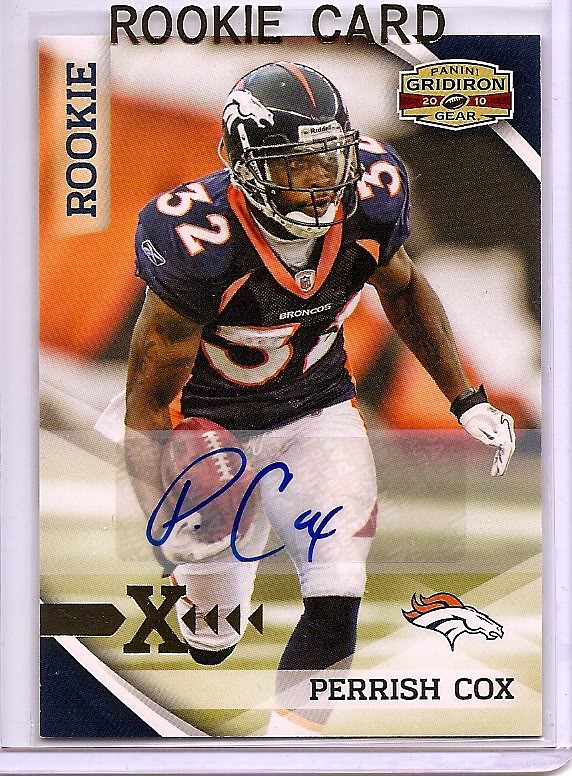This image features a detailed rookie trading card of football player Parrish Cox. The card has an orange and green blurred background with an additional black and striped pattern. Parrish Cox, wearing a blue Broncos uniform with white pants and number 32 emblazoned on his shoulders, is depicted running and holding a football in his left hand. His black helmet prominently displays a horse logo with an orange mane. The top of the card is labeled "Rookie Card" in black, and "Rookie" is also written vertically on the left side. The lower section of the card displays Parrish Cox's name. Additionally, a large letter 'X' and a Denver Broncos logo can be seen to the left and bottom right, respectively. The card is framed by a silver band, with the inscription "Panini Gridiron 2010 Gear" also present, marking it as a collectible item from that series.